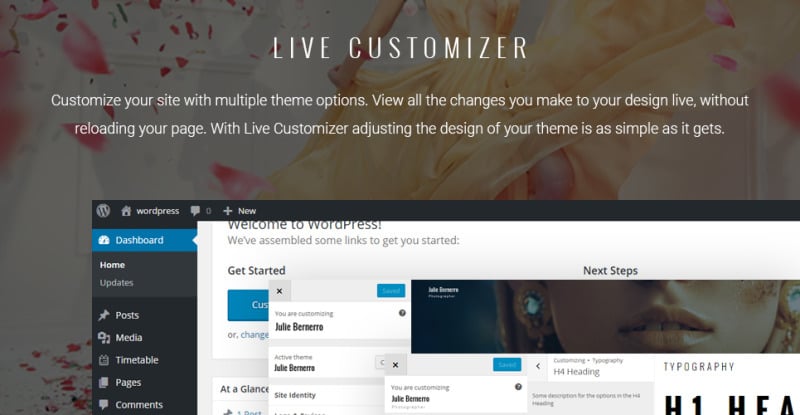The image features a section of a website with a visually captivating background. Dominating the background is a partial view of a woman from the chest down, dressed in a flowing outfit adorned with pink floral patterns, seemingly caught in a moment of dancing or twirling. The motion causes the dress to lift gracefully at the sides, emphasizing its delicate design. The backdrop is predominantly dark, which beautifully contrasts with the light-colored floral print.

Overlaying the background is a prominent white text heading in all capital letters that reads "Live Customizer." Below this, in smaller white print, the text elaborates: "Customize your site with multiple theme options, view all the changes you make to your design live without reloading your page. With Live Customizer, adjusting the design of your theme is as simple as it gets."

At the top edge of the image, there is a black banner with the white WordPress logo. The dashboard menu is highlighted in blue, featuring various sections such as Home, Updates, Posts, Media, Timetable, Pages, Comments, among others. Below the dashboard heading, the text states, "Welcome to WordPress, we've assembled some links to get you started," followed by a "Get Started" button. The section continues with a "Next Steps" heading and indicates "You are customizing active theme site identity."

This detailed interface showcases the customization capabilities provided by WordPress, emphasizing the user-friendly nature of designing and adapting website themes with the Live Customizer tool.